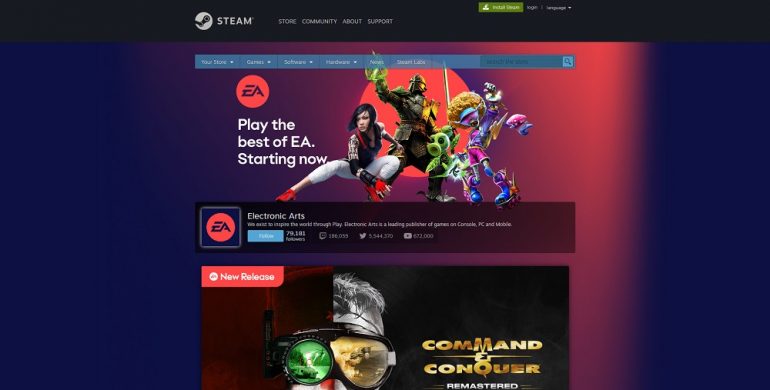The image appears to be a screenshot from the Steam website. At the top, prominent sections like "Store," "Community," "About," and "Support" are visible, along with the Steam logo. 

In the main section, there is a banner promoting EA Play, featuring the tagline "The Best of EA Starting Now." The banner showcases various video game characters:

1. A female character with black hair, wearing white pants, red gloves, black armbands, and red heels.
2. A male character dressed in armor that has a samurai-space theme, wielding a greenish sword.
3. A skateboarding kid character with robot-like features, including purple and pink hair with green highlights, and wearing goggles.

Below the banner, Electronic Arts displays their traditional red EA logo with text likely related to their social media links and other information.

Towards the bottom of the image, there is a highlight for a new release: the remastered edition of "Command and Conquer." The promotional image features a male figure with asymmetrical goggles, where one goggle shows green and yellow war imagery.

The entire setup is set against a reddish-blue background, adding a striking visual contrast to the Steam store interface. Above the EA Play banner, there are additional navigation options for "Store," "Games," "Software," and a search bar, indicating the comprehensive offerings available on the platform.